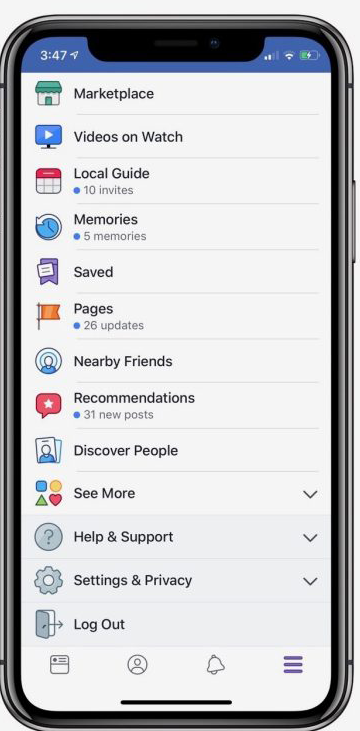The image showcases a detailed close-up shot of a sleek smartphone. The device, rendered in metallic material, exhibits a shiny outer surface with visible reflections along its curved edges and bottom. The screen displays a menu rich with a variety of options against a clean white background, segmented by single-pixel grey lines. The status bar at the top indicates it is 3:47 PM, with a light blue header. Signal strength is at 2 out of 4 bars, Wi-Fi connectivity at 2 out of 3, and the battery level sits at approximately 50%.

Beneath the status bar, various menu options are listed with corresponding icons to their left. The first option features a storefront icon with a green roof labeled "Marketplace." The next option shows a computer screen with a white play button in a blue field titled "Videos on Watch." Following this is a calendar icon with a red header named "Local Guide" and a blue dot indicating "10 invites." An icon of a clock with an arrow going counterclockwise represents "Memories," showing a count of five. A purple bookmark icon displays "Saved," and an orange flag icon signals "Pages," highlighting 26 updates. 

A profile icon with a beacon signifies "Friends Nearby." A red speech bubble with a star highlights "Recommendations," with 31 new posts. Additionally, lanyard icons suggest "Discover People," and options at the bottom include "See More," represented by a blue square, a triangle, and a heart. The final section of the menu offers straightforward navigation with options labeled "Help," "Support," "Settings," and "Logout," concluded by a simple navigation menu at the bottom.